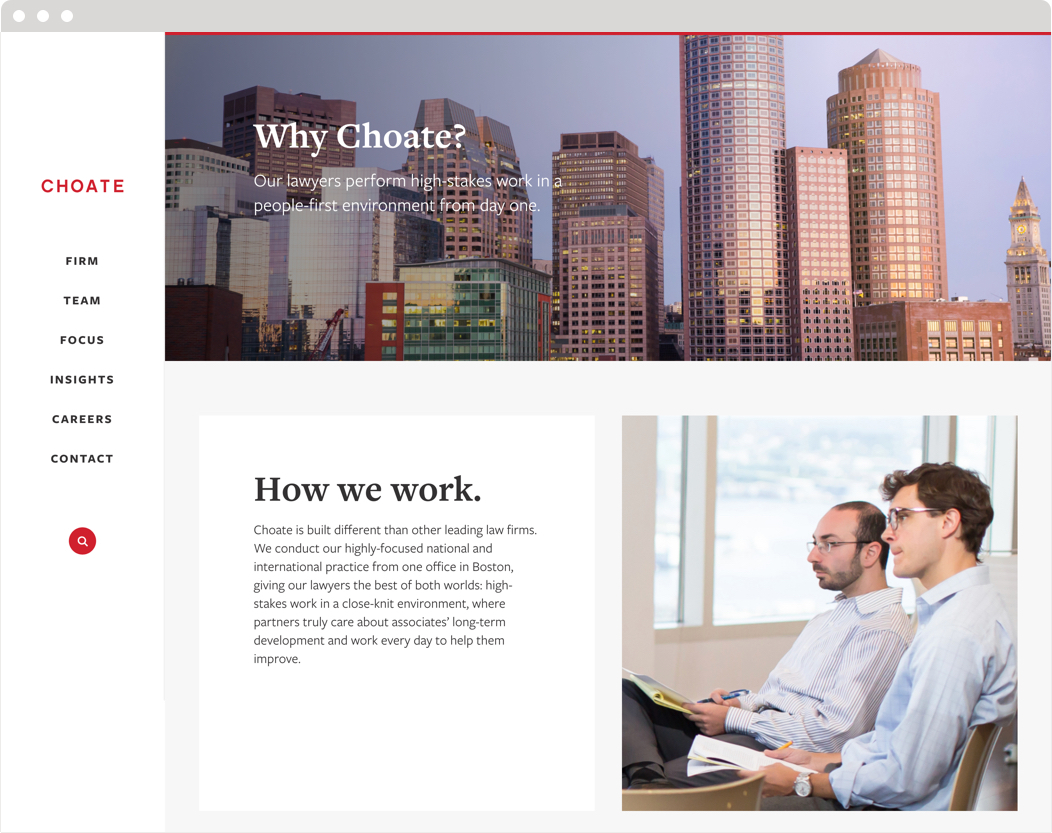Homepage of Choate, Hall & Stewart LLP's Website

At the top of the webpage, there's a gray border with three white dots. To the left is a white section featuring the name "Choate" in red. Below this header are navigation tabs labeled: Firm, Team, Focus, Insights, Careers, and Contact. A red search icon is also placed beneath the tabs. The main section displays an image of a business district skyline, indicative of office buildings. Overlaid on this image, large text reads, "Why Choate? Our lawyers perform high-stakes work in a people-first environment from day one."

Below the main text is a section titled "How We Work," accompanied by a short write-up. To its right, there is an image of two men sitting in chairs with backrests inside an office, intently focusing on something. The presence of a window shows that it’s daytime outside. The accompanying text explains, "Choate is built differently than other leading law firms. We conduct our highly focused national and international practice from one office in Boston, providing our lawyers with the best of both worlds: high-stakes work in a close-knit environment where partners genuinely care about associates' long-term development and work daily to help them improve."